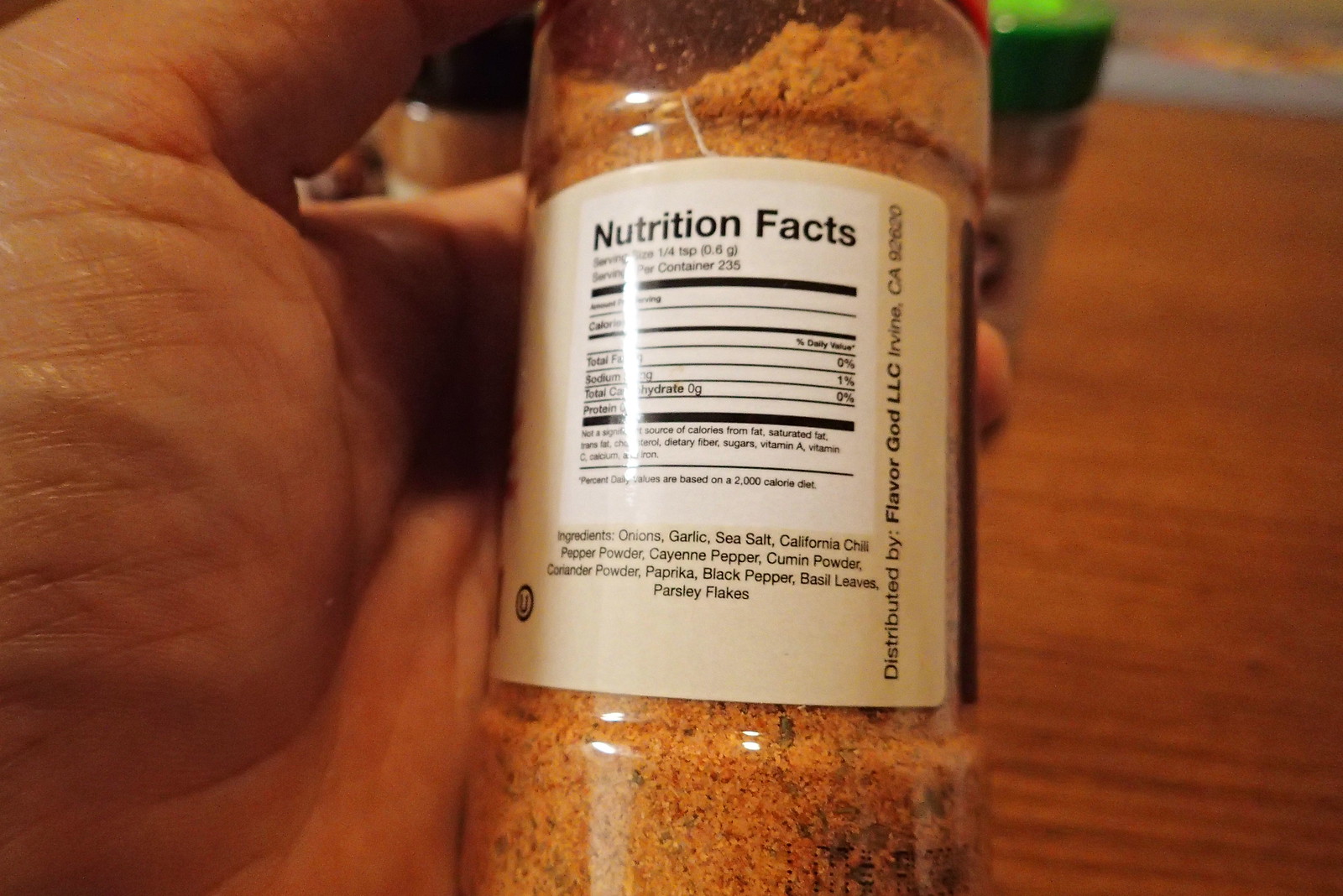In the image, a white man's left hand is holding a brown bottle of mixed seasoning, clearly showcasing the red lid and the seasoning within, which appears orange with green and yellow specks. The label, showing nutritional facts, is blurry due to a light glare, making specific details like calorie and fat content hard to decipher. The ingredient list includes onions, garlic, sea salt, California chili pepper powder, cayenne powder, cumin powder, paprika, black pepper, basil leaves, and parsley flakes. The bottle is distributed by Flavor God LLC, Irvine, California. In the background, a brown wooden counter is visible, with additional spice bottles—one with a green lid and another with a black lid—positioned behind the hand.